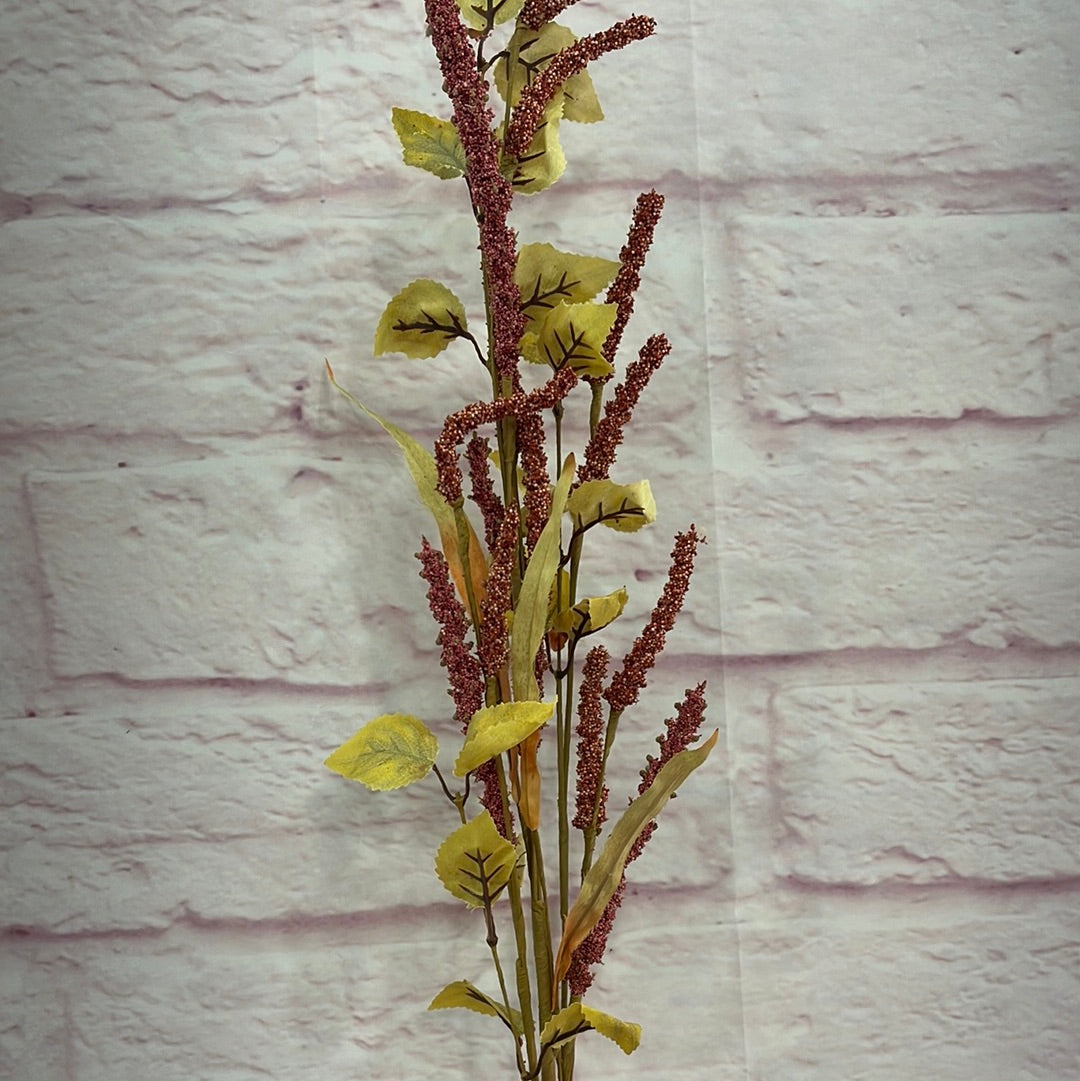The photograph captures a tall plant positioned centrally in an indoor setting, framed against a white painted brick wall that has a subtle pink tinge and minor gouges that have been painted over. The plant's slender green stems rise vertically from the bottom of the image and continue out of the top frame. It features light green, tapered leaves that resemble blades of grass, some of which display a vein-like black structure. Scattered along the stems are elongated, tubular red blossoms, arranged horizontally and appearing somewhat fuzzy. There are approximately eight or nine of these vibrant flowers, grouped in clusters. The plant casts a shadow on the wall, likely from the camera's flash, enhancing the texture and depth of the scene. The wall's brick pattern adds a rustic backdrop, while the overall composition exudes an intricate blend of natural and artificial elements, making it hard to discern if the plant is real or synthetic.